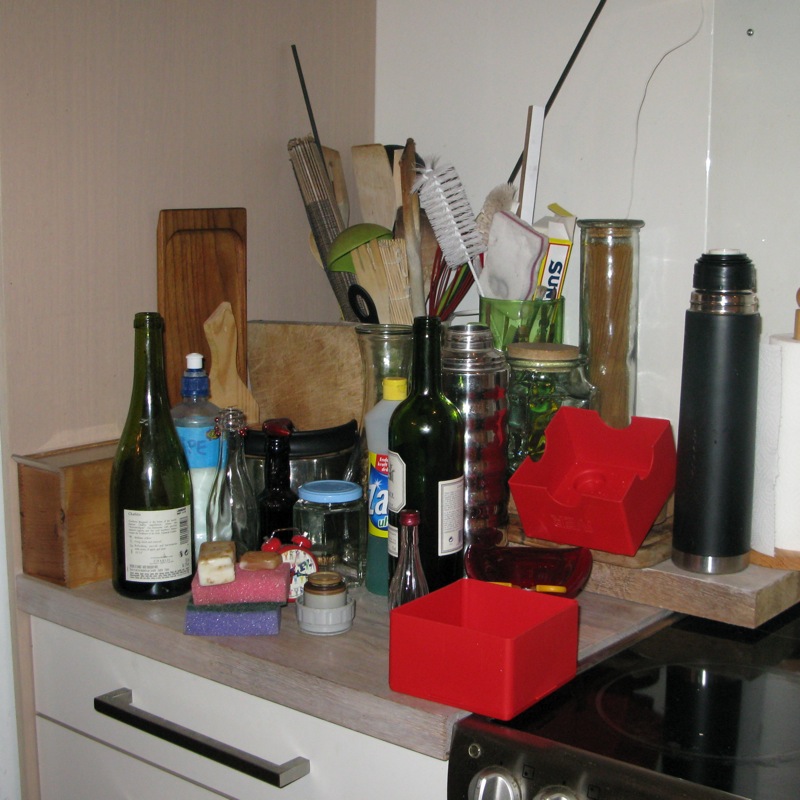This photograph captures a cluttered corner of a kitchen, identifiable by a drawer beneath a cupboard and a stovetop visible in the bottom right corner. The space is filled with a variety of items, contributing to a messy and chaotic appearance. There is an unlabeled bottle, along with two sponges. Red containers that resemble children's stacking blocks are strewn about. A wooden cutting board stands against the backdrop, accompanied by a cleaning solution and an empty glass container, possibly a wine bottle. 

In the background, several items are arranged on what appears to be a wooden block. These include a water bottle and a tall, transparent container filled with uncooked noodles. Next to this is another glass container, potentially a margarita cocktail shaker, though its contents are unclear. Further back, there are two additional glass containers, likely vases, holding an assortment of wooden spoons, cleaning products, and yet another sponge. The scene resembles a collection of assorted items that have been haphazardly placed on the counter, possibly during a decluttering effort. The overall impression is one of disarray, with a mix of kitchen-related and unrelated objects scattered around.